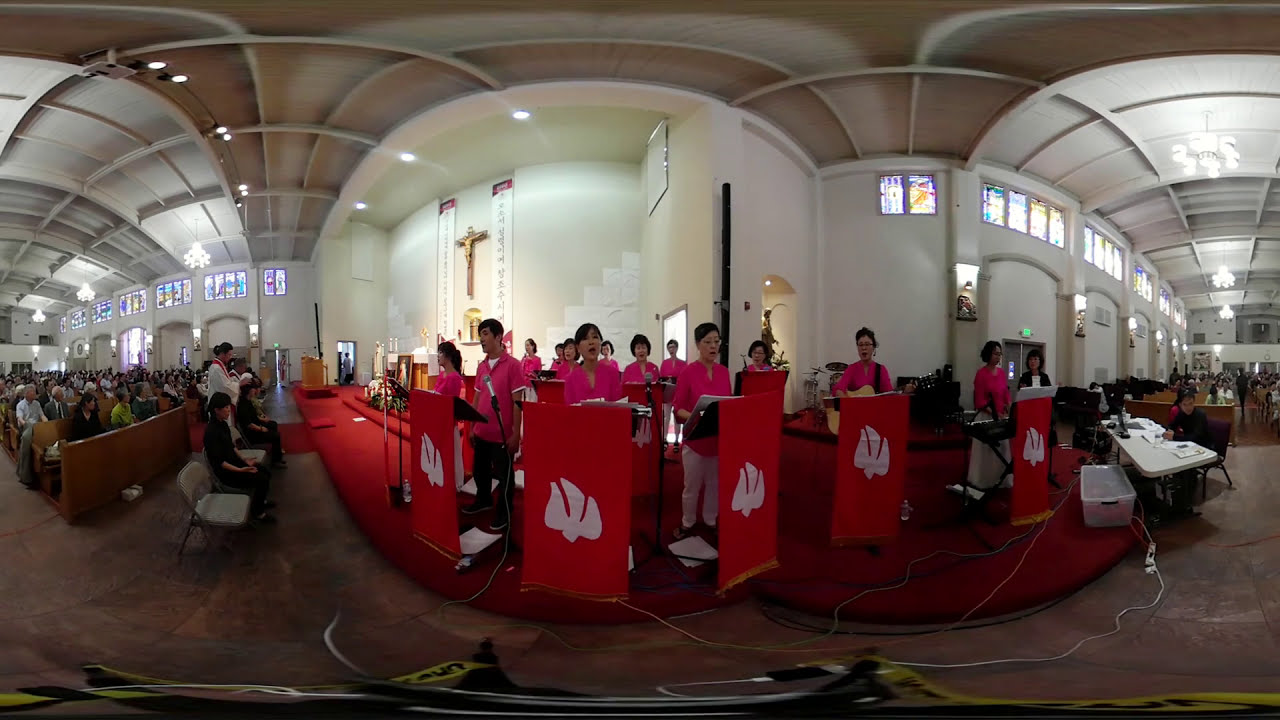In this fisheye-lens-distorted image, a group of Asian individuals wearing pink shirts are positioned on a stage, apparently singing behind podiums covered with red rectangular banners displaying a white three-sectioned leaf logo. Each person has a microphone and note carriers in front of them. The setting is a church, evidenced by a large golden cross on the left wall and rows of pews filled with congregants. The left side of the image shows people standing and pews crowded with seated individuals, with one empty chair prominently in front. To the right, a light-colored table has several people seated around it. The curved, arching white walls and ceiling are adorned with stained glass windows near the top, creating a dramatic, warped effect due to the lens. White cords run along the floor, likely connecting to the microphones, further contributing to the detailed depiction of this church service scene.